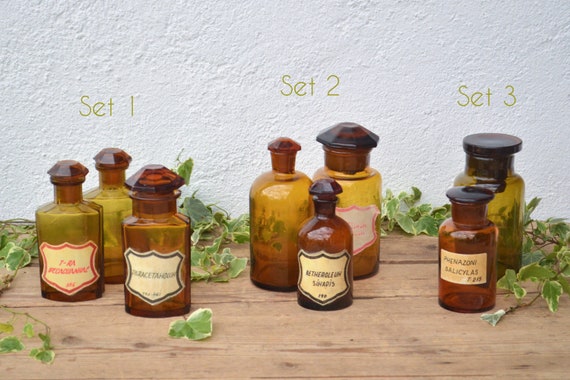This detailed color photograph captures a collection of small, antique-style glass bottles of varying colors, primarily orange, with some appearing brown and yellow. These bottles are carefully arranged in three distinct sets on a wooden surface against a white plaster wall. Each set is distinctly labeled from left to right as "Set One," "Set Two," and "Set Three." The first and second sets each have three bottles, whereas the third set features two bottles. Some of the bottles have shield-shaped labels, although the text is too pixelated to read clearly. One label on the rightmost bottle of the image partially shows the word "SALICYLAS," suggesting they might contain chemicals or old prescriptions. The bottles all feature glass stoppers and exude a vintage apothecary vibe. Additionally, there are ivy leaves scattered in the background, adding a touch of greenery to the scene.